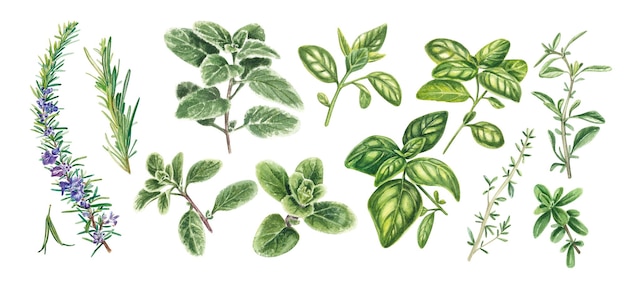The image displays a collection of various plant leaves and stems set against a white background. On the left side, a long stem adorned with green leaves and delicate purple flowers protrudes upwards. Another similar stem with only green leaves runs parallel to it. To their right, a mid-height stem features oval-shaped leaves organized symmetrically along its length, culminating in larger foliage at the base. Adjacent to this is a striking leaf with both a dark and light green coloration, prominent veining, and V-shaped patterns. Further to the right, a basil-like leaf is depicted alongside a couple more sprigs with tiny leaves. This detailed assembly of diverse plants appears bright and vibrant, with varying shades of green and occasional hints of yellow and purple flowers. The leaves vary in size, shape, and color, contributing to a dynamic and colorful composition that suggests a somewhat animated or cartoonish style. The plants are organized in two rows, each containing about five to six distinct sprigs.